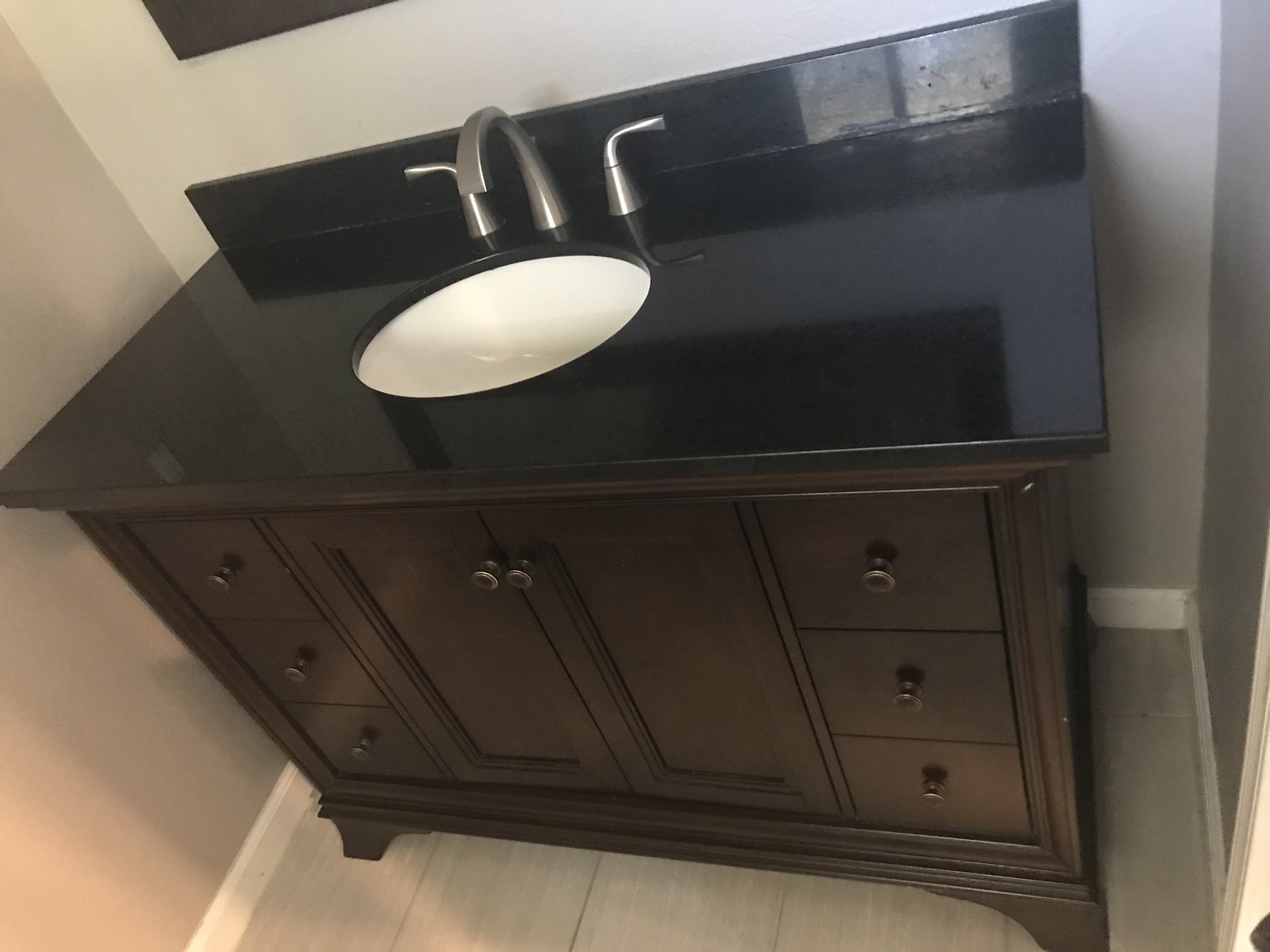This photograph depicts a guest bathroom with a centrally featured white basin set into a black countertop, complemented by a small black backsplash. The countertop, stretching nearly wall-to-wall, is supported by a dark walnut wooden cabinet. The cabinet has distinctive round handles on its cupboard doors and round knobs on each of its six drawers, arranged three on each side. The room's floor consists of grey, rectangular tiles, paired with white skirting. The walls are painted in a matching grey hue, enhancing the room's cohesive aesthetic. Above the basin, a large brown-framed mirror, matching the cabinet's finish, occupies the back wall. The reflection in the backsplash suggests the presence of a window behind the photographer. The door frame is visible in the bottom right corner, indicating the photo was taken from the doorway. Overall, although the room is not brightly lit, the well-coordinated design elements are evident.